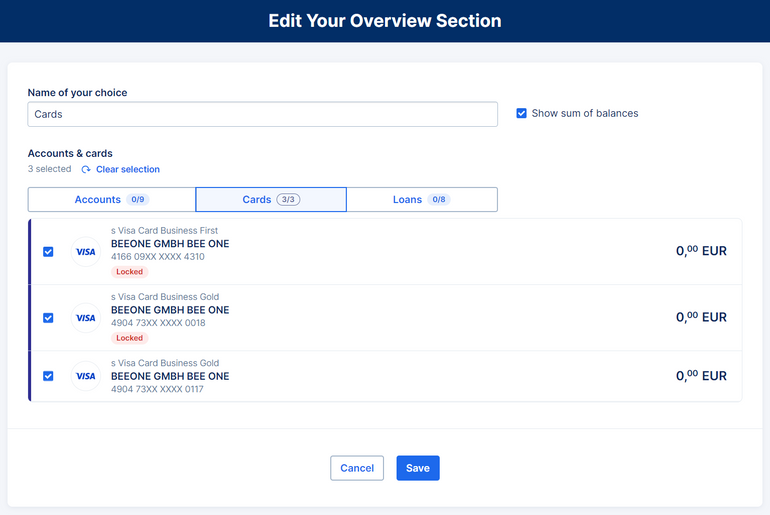Screenshot Description: 

The image displays a user interface screen with a predominantly white background and multiple information boxes in varying shades of blue. At the top, there is a navy blue box containing the text "Edit your overview section." Below, another navy blue box reads "Name your choice," next to which is a white text field filled with the word "Cards." Beside this text field is another smaller blue box labeled "Show some balances" with a checkmark inside.

Further down, details of selected financial accounts and cards are presented:

- "Accounts and cards: three selected"
- "Accounts: 0 out of 9"
- "Cards: 3 out of 3"
- "Loans: 0 out of 8"

Three Visa business cards are listed, all from the same bank, B1 GMBHB1:
1. **Visa Business Card in blue**: Marked with a blue check square, showing a balance of "0 euros."
2. **Visa Business Card in gold**: Marked with a blue check square, showing a balance of "0 euros."
3. **Visa Business Card in blue**: Again marked with a blue check square, labeled "Visa Card Business Gold," revealing a balance of "0 euros."

At the bottom of the screen, two buttons are visible: "Cancel" on the left and "Save" on the right, with "Save" highlighted in a blue box, implying the user's current intention to finalize the changes.